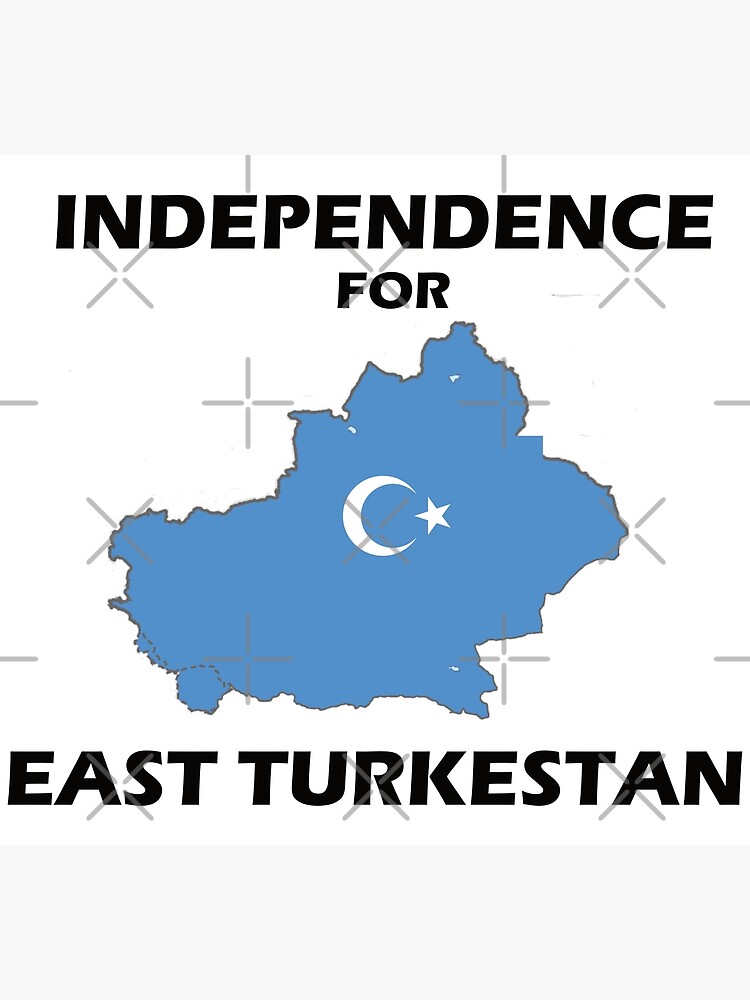This is an image of a poster advocating for the independence of East Turkestan. Dominating the poster is a blue-shaded outline of the country, bordered in dark gray against a plain white background. Inside the blue silhouette of East Turkestan, there's a prominent crescent moon and a star, likely representing the region's flag. Bold text at the top declares "Independence for East Turkestan." Additional elements on the poster include small black symbols resembling crosses and X's, possibly indicating map coordinates or other geographical markers, though their specific meanings are unclear due to the small size of the writing. The overall design seems computer-generated, focusing on a clear and strong visual message for the political cause.